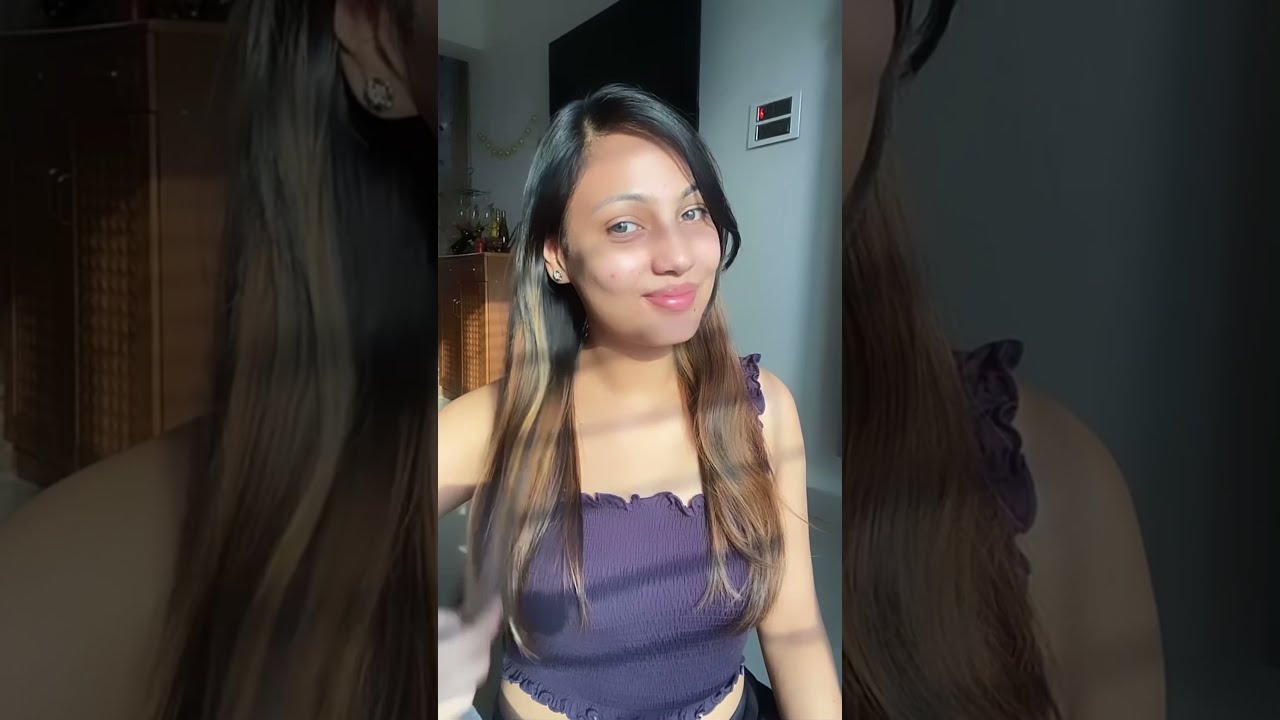The image is a horizontally rectangular photograph with grayed-out areas on either side, featuring a more narrow vertical center image of a young woman in her late teens, around 18 or 19 years old. Her straight hair transitions from black at the roots to dirty blonde at the tips, and it is parted on the side, cascading well past her breasts. The young woman is smiling warmly, with her head and body slightly tilted to the right, revealing pink lipstick on her lips. She's wearing a purple crop top that leaves her shoulders bare and covers just her midsection, revealing some of her midriff. Behind her, the white walls of the room are visible, along with a dark doorway to the right and a wicker cabinet with some bottles on top to the left. Above the cabinet hangs a small banner, though its details are indistinct. Light shines through a window, casting pale stripes of shadow across her body. On the right and left sides of the central image, the photograph is blown up and darkened, focusing on close-ups – the left side features her hair falling over her shoulder and a visible earlobe with a small earring, while the right side emphasizes her right shoulder and the flowing strands of her hair. The photograph captures her from the waist up against this softly detailed backdrop.